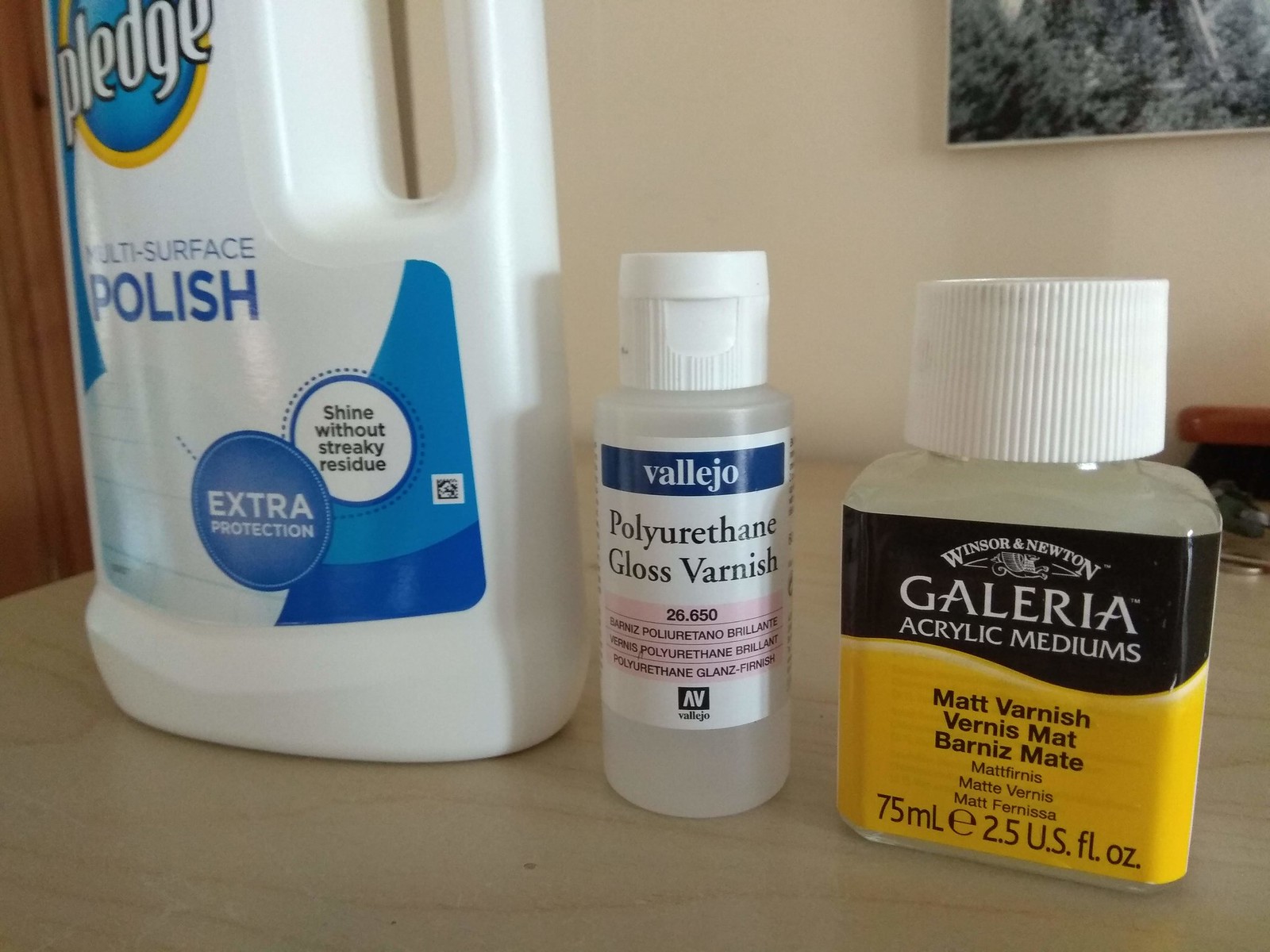The detailed close-up image showcases three containers on a light wood-colored table, with a tan wall and part of a picture with gray and black hues visible in the upper right corner. On the upper left, there's a dark wood area, likely a door. The foreground features three distinct products:

1. On the left, a large white bottle of Pledge Multi-Surface Polish with a cut-off top, displaying blue text with highlights like "extra protection" and "shine without streaky residue" in different circles.
2. In the center, a small clear cylindrical container with a white flip top labeled Vallejo Polyurethane Gloss Varnish, with additional multilingual text.
3. To the right, a wider, shorter rectangular container with a white screw top labeled Windsor & Newton Galleria Acrylic Mediums Matte Varnish, detailed with its volume of 75 milliliters (2.5 US fluid ounces).

The detailed and neatly arranged labels and varied shapes of the containers stand out against the light wood and muted background elements.